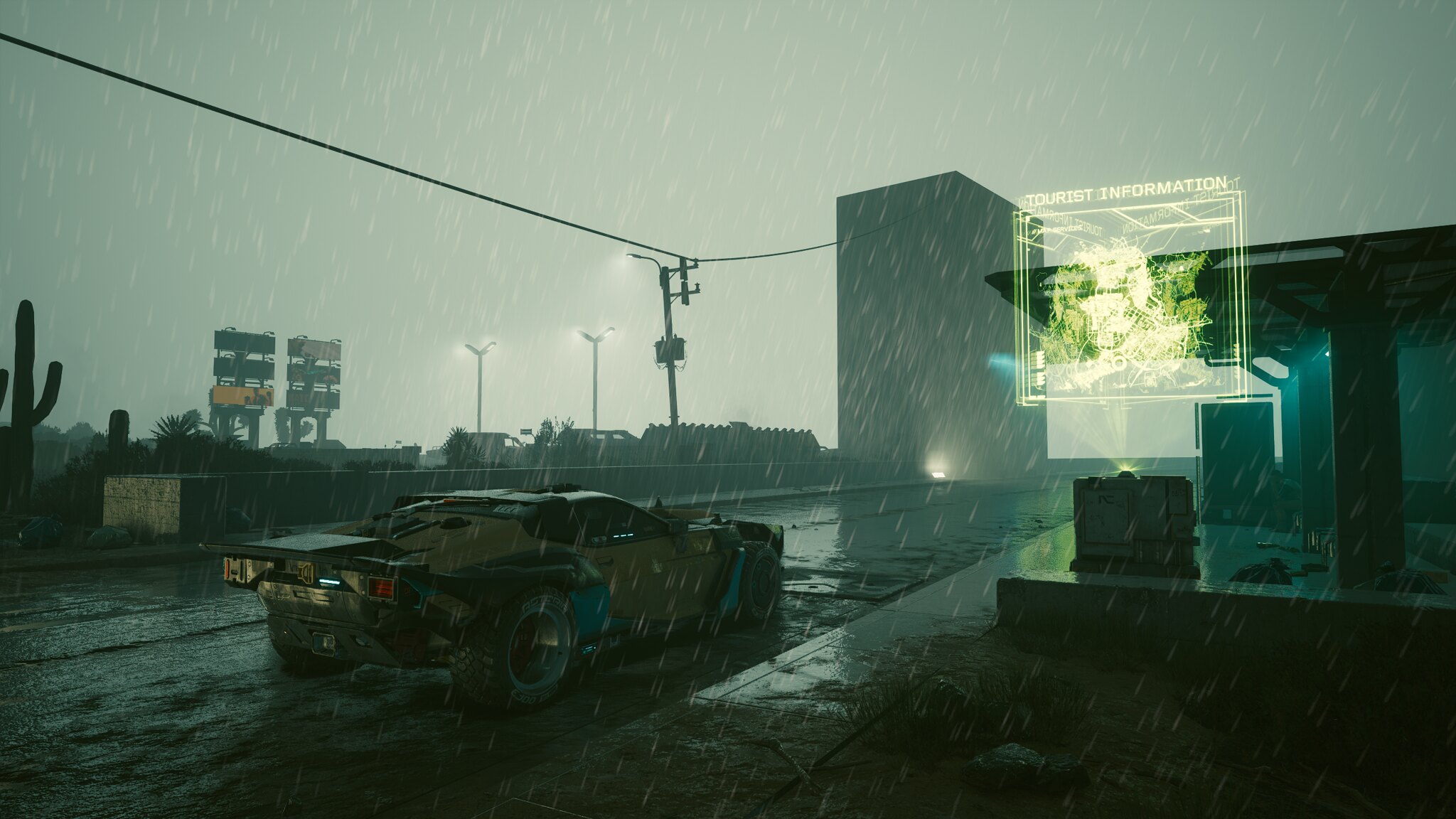This detailed image appears to be a highly stylized 3D render or an in-game screenshot, set in a dystopian, rain-soaked street within a desert environment. The scene is dominated by a heavy downpour, with rain visibly falling and pooling on the road. The sky is overcast with a very grey and ominous hue, enhancing the dramatic atmosphere. 

On the left side of the image, several cacti and desert shrubs stand out, juxtaposing the arid landscape with the rain-soaked street. Dominating the center of the road is a futuristic car that has a distinct cyberpunk aesthetic, characterized by its sharp design, thick tires suitable for off-road terrains, and a striking paint job with yellow and blue trim.

On the right side, there is a holographic display projecting tourist information in bright neon green and yellow hues, adding a science-fiction element to the setting. The background reveals a tall, windowless building, and illuminated streetlights, which suggest that it is nighttime. The streetlights, along with a pole carrying what might be a traffic signal, hint at urban infrastructure that contrasts with the otherwise barren desert surroundings. This captivating blend of futuristic elements and natural scenery makes for a visually compelling and immersive scene.